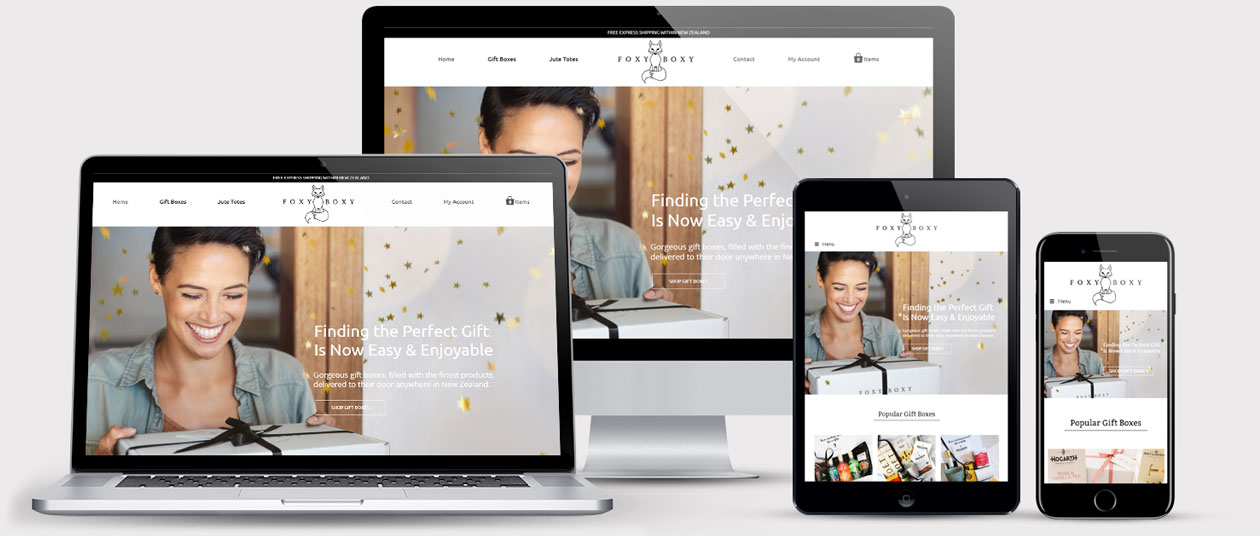This cropped desktop screenshot showcases a versatile e-commerce website named "Foxy Boxy" displayed on four different devices, presumably older Apple models including a MacBook, iMac, iPad, and iPhone. The pale industrial gray background provides a stark contrast to the vibrant, user-friendly website design. The website features a whimsical cartoon fox logo and a clean, white interface with navigational tabs labeled Home, Gift Boxes, Juice Totes, Contact, My Account, and Items.

Prominently displayed is an image of a cheerful woman with short dark brown hair and a radiant smile, dressed in a denim jacket. She holds a white gift box adorned with a sleek black ribbon. The backdrop of the website image is adorned with golden star-shaped confetti, creating a festive atmosphere. An inviting tagline in white text reads: "Finding the perfect gift is now easy and enjoyable. Gorgeous gift boxes filled with the finest products delivered to their door anywhere in New Zealand." 

The screenshot highlights the compatibility of the "Foxy Boxy" website across multiple devices, underscoring the platform’s accessibility and user convenience, irrespective of the device being used.